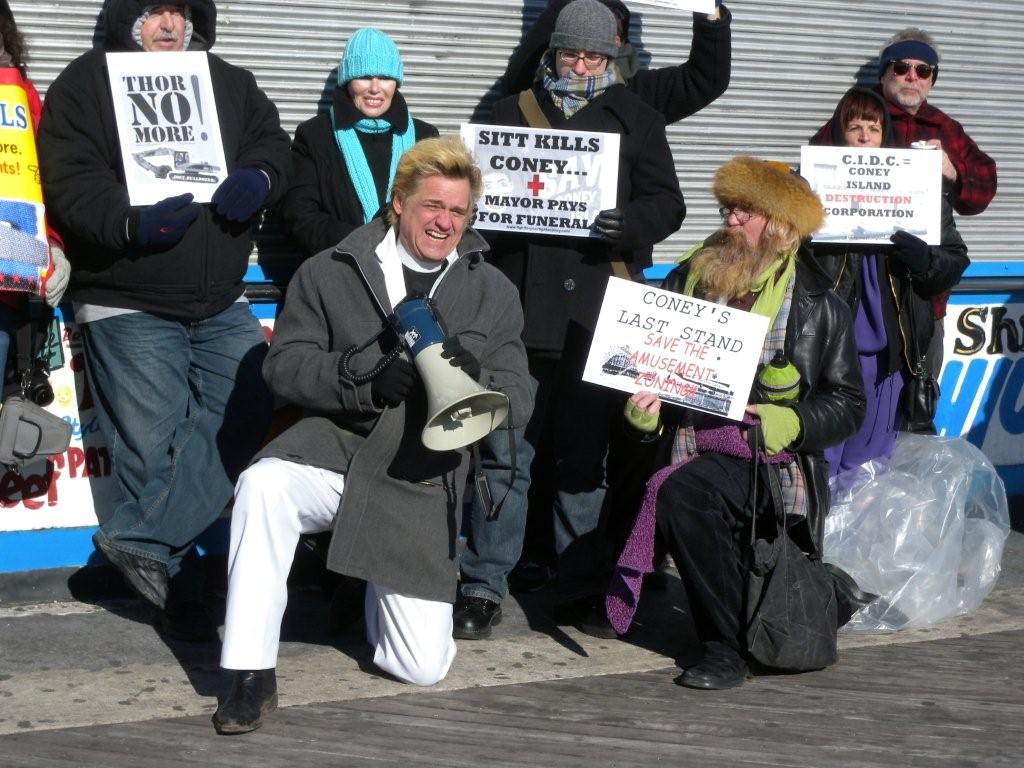The image captures a serious outdoor protest set in regular daylight. A diverse group of men and women, bundled in heavy winter clothing, are gathered on a sidewalk adjacent to a curb with a road in front of it. They appear to be standing in front of a metal building adorned with some kind of signage that is partially obscured. 

At the forefront of the scene, an older man with blonde hair, dressed in white pants and a gray jacket, is kneeling and holding a megaphone. He is flanked by another man with a long blonde beard. Surrounding them, protesters are holding up various white signs with bold messages that underscore their grievances: "Coney's Last Stand," "Save the Amusement Zoning," "Thor No More," "Sit Kills Kony," "Mayor Pays for Funeral," and "CIDC Kony Island Destruction Corporation." The atmosphere and the attire of the protesters suggest a sense of urgency and resolute opposition to recent developments concerning Coney Island.